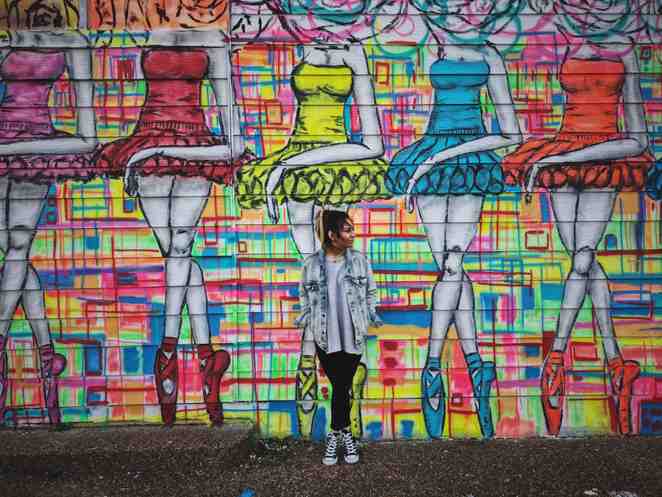A woman is leaning against a colorful, artistically spray-painted graffiti wall, featuring five ballerina dancers gracefully poised on their toes. The woman, who has dark hair with yellow highlights, is dressed in a light blue jean jacket, a white shirt, black pants, and black and white Chuck Taylor sneakers. She stands on a gray, gravel-like ground with specks of white. 

Each ballerina is vividly depicted in different colors: the one on the far left is adorned in a purple dress with matching shoes, followed by a ballerina in red, the middle dancer in yellow, the next one in blue, and the final dancer in orange. Their left arms are elegantly crossed over their waists. The background is a lively mosaic of squares and rectangles in shades of blue, orange, red, green, and white, creating a dynamic and vibrant scene. The woman's contemplative pose and the surrounding splashes of color make the image an eye-catching display of urban art.